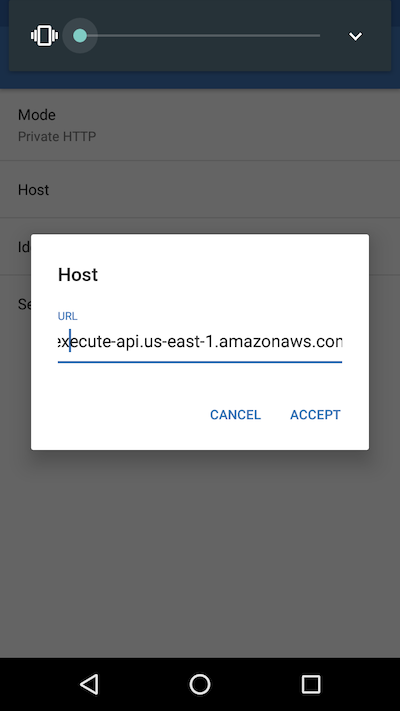The image appears to depict a cellphone screen with a user interface for an API execution tool. In the background, on the top left corner, there is a white vibrate icon, indicating that the phone is on vibrate mode. Below this icon, there is a slider bar that has been moved all the way to the left. On the right side of the screen, a pull-down menu indicator is visible.

The entire background is grayed out, overlayed with a prominent white rectangular box that is horizontally elongated. In the top left corner of this box, the word "Host" is displayed, followed by a field labeled "URL." The URL field contains the text "https://api.us-east-1.amazonaws.com," indicating an endpoint for an API service. A blue cursor is positioned within the text, specifically between the "x" and "e" in "execute."

Beneath the URL field, there are two blue action buttons labeled "Cancel" and "Accept."

Below this white rectangle, into the grayed out background territory, there is a blue strip followed by a white background section containing the text "Mode: Private HTTP." A gray line underneath this text demarcates a new section. The word "Host" also appears here, followed by another gray line.

Further below, another section is partially visible, displaying the text "ID" and part of another line initiating with the letter "S." The rest of the information is obscured and not discernible.